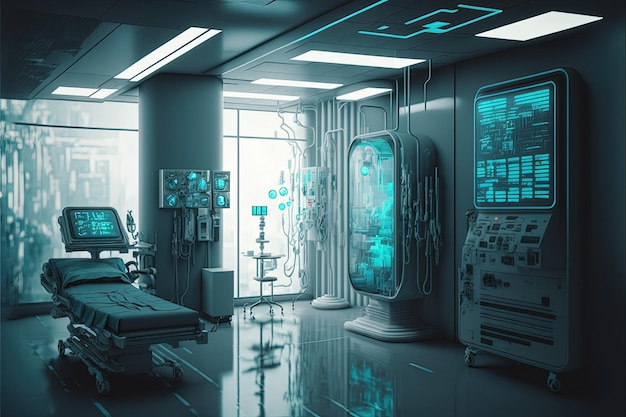This image depicts a futuristic, high-tech hospital room that feels straight out of a science fiction movie set in the year 2500. Central to the room is a compact, movable hospital bed complete with an armrest, suggesting advanced ergonomic design. Attached above the bed is a laptop-screen-sized monitor displaying green numbers, letters, and symbols, likely for vital statistics such as blood pressure and oxygen saturation. The room is bathed in a blue ambient light, contributing to its futuristic aesthetic, while white lights accentuate the high-gloss, reflective flooring.

Facing the bed on the far wall, two large machines dominate the space. The machine closest to the camera features a sizable green and black display with multiple green blocks, potentially representing intricate data or patient diagnostics. The adjacent machine, adorned with various tubes, appears to be equipped for IVs and other medical infusions. Adjacent to these machines, pillars in the room feature numerous little LED readouts, whose functions remain unclear but add to the high-tech feel.

In addition, a roll-around cart with an LED screen sits by the pillar, hinting at mobility and flexibility in the room's medical capabilities. There's also the intriguing suggestion of a doorway-like machine, which could be a futuristic healing chamber, adding an element of speculative technology to the setting. A window provides a view, though it's ambiguous whether it looks out onto the outdoors or into another room. The absence of people sharpens the focus on the advanced technological environment, making it a quintessentially futuristic medical station.